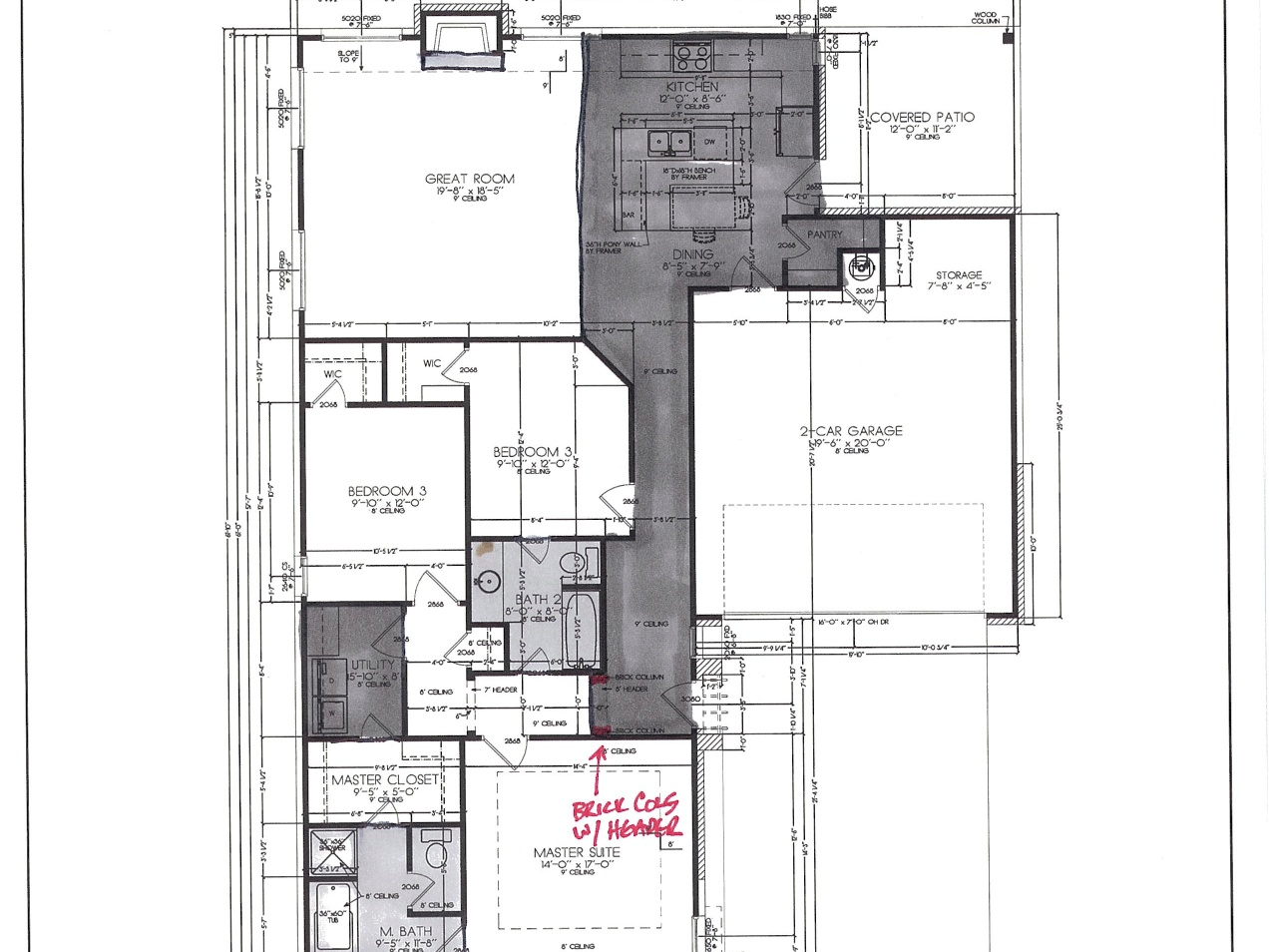This sketch depicts a detailed floor plan of a house. The blueprint includes several key areas, delineated by lines of varying significance. Vertical lines run throughout the layout, with four prominent lines in a row, separated by a space, and an additional line indicating the house's exterior walls. Different colored lines denote window placements.

On the top left of the sketch is a large square space labeled as the "Great Room," adjacent to which is the kitchen, also marked as a square. Connected to the kitchen is an L-shaped pantry, and extending from the kitchen is a small dining area. Nearby, there is a square space designated as the covered patio. Moving to the right of the kitchen, there is a hallway leading to various rooms.

On the right side of this hallway, there is a substantial square space allocated for a two-car garage. Along the hallway are three bedrooms. The master suite, represented as a square, features a master closet and a master bath. Adjacent to the master suite are Bedroom Two and Bedroom Three. Between Bedroom Three and the master closet is a small square utility closet. Additionally, there is another bathroom located along this hallway.